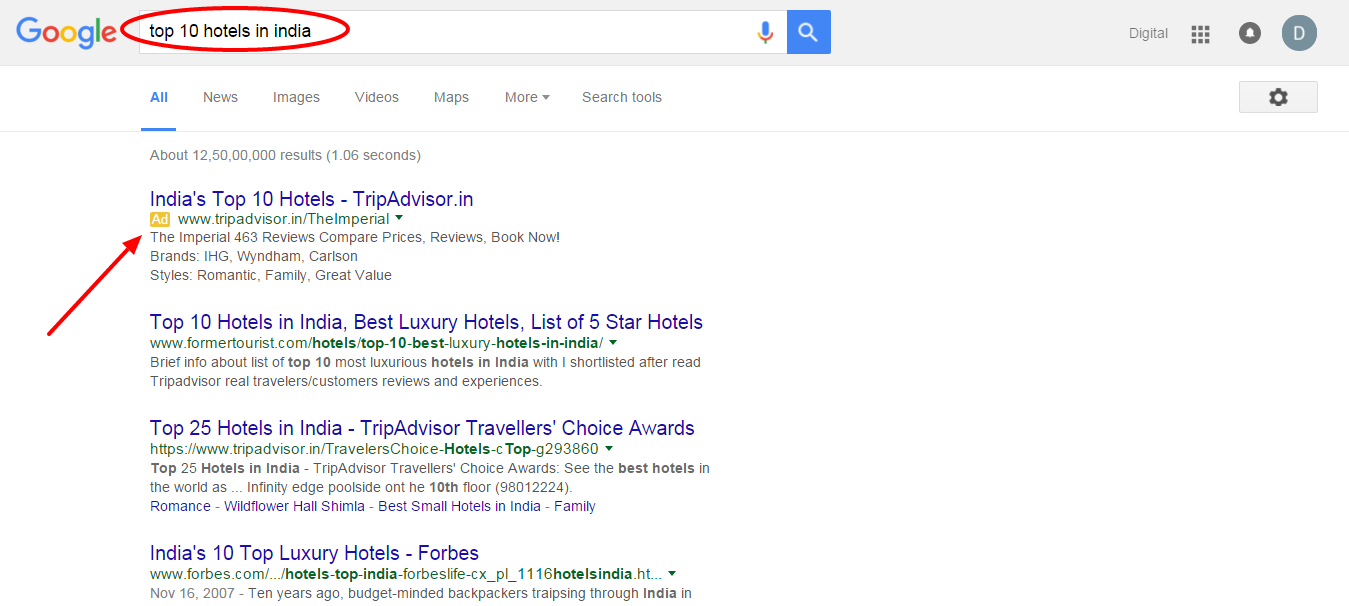The image showcases a Google search results page. At the top, the iconic Google logo is displayed within a gray rectangle, featuring the signature blue, red, yellow, and green colors. In the search bar, highlighted with an oval red circle, are the words "Top 10 Hotels in India." 

Below the search bar, the first search result is titled "India's Top 10 Hotels." A red arrow points to this result, which is presented in blue text as "India's Top 10 Hotels Trip Advisor." Beneath this, a paragraph highlights "The Imperial," featuring 463 reviews along with options to compare prices and book instantly.

Further down, another search result is titled "Top 10 Hotels in India Best Luxury Hotels List of 5 Star Hotels," also in blue text. This title is followed by a brief introductory paragraph giving an overview of the top 10 hotels, with additional details accessible via a click.

The next result is titled "Top 25 Hotels in India Trip Advisor Traveler's Choice Award," in blue text, followed by a descriptive paragraph. At the bottom, there is a mention of "India's Top 10 Luxury Hotels Forbes."